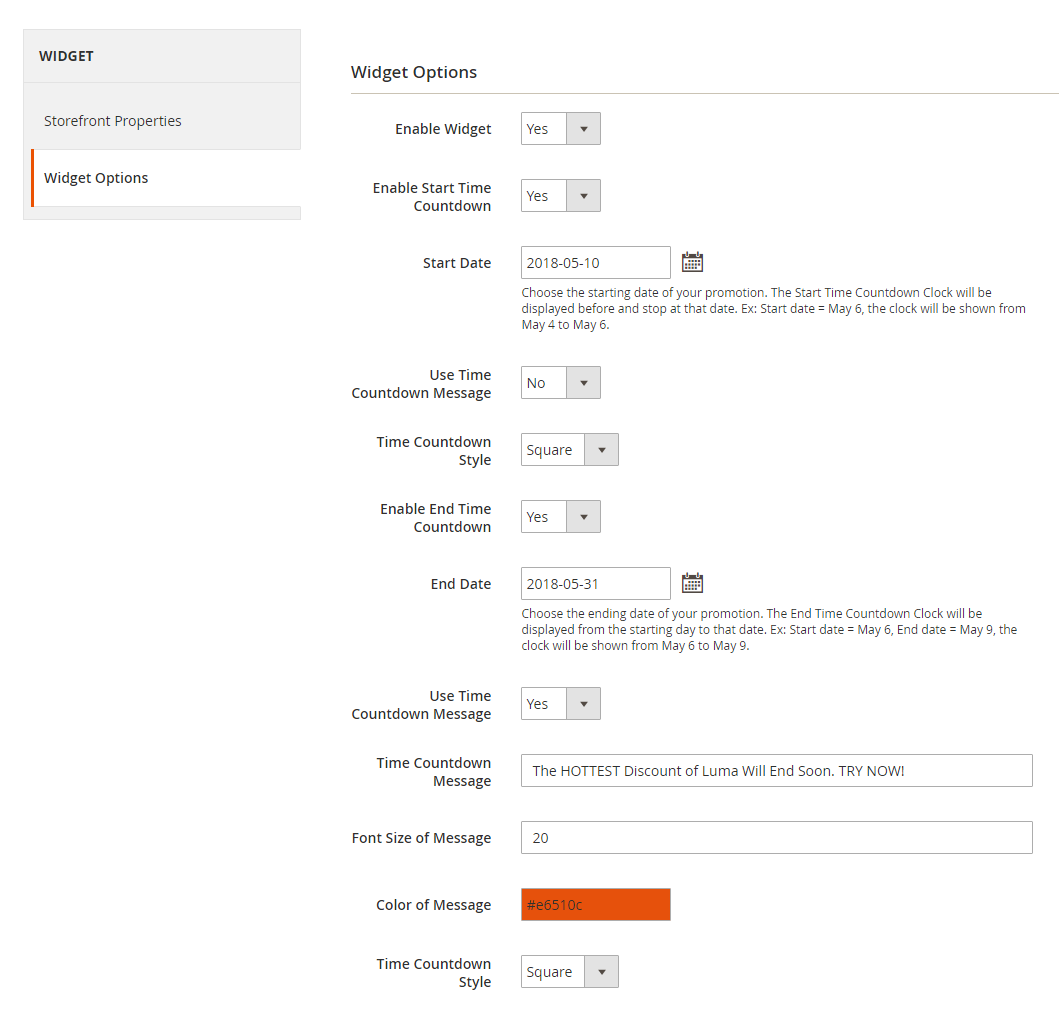This screenshot captures a user interface for managing widget settings. On the left-hand side, there's a gray sidebar featuring several options. At the top, "Widget" is written in gray text. Below that, "Storefront Properties" is listed, and beneath it, highlighted in white, is "Widget Options," marked by a red vertical line. Selecting "Widget Options" displays various settings.

The central area details several customization fields starting with "Enable Widget," which has a toggle option set to "Yes." Next is "Enable Start Time," which is also enabled with a "Yes" option. Under this, a small calendar icon allows the user to pick a start date, providing a clear visual representation. There's a setting for "Use Time Countdown Message" with an option to select "Yes" or "No" via a drop-down arrow.

Moving down, the form includes an "End Date" section followed by a paragraph field for the time countdown message. In this example, it reads, "The hottest discount of Luma will end soon. Try now." Text customization options come next, where the font size is set to "20" and the color of the message is specified through a red hex code. The "Time Countdown Style" is selected as "Square," accompanied by a gray box with an arrow.

This detailed configuration setup allows users to tailor widget parameters effectively, ensuring customized and timely promotional content displayed on storefronts.